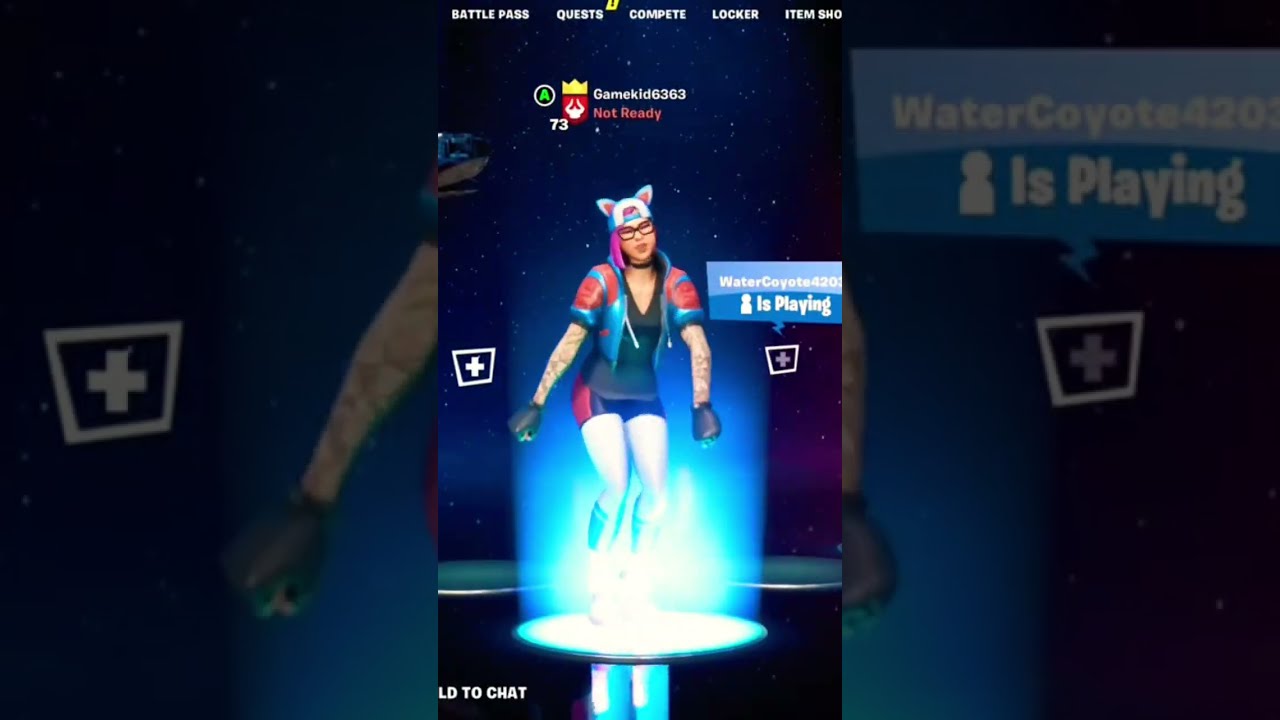The image depicts the start of a video game on a cell phone, shown in a rectangular horizontal format with a very dark background. Portions of the left and right sides are grayed out and somewhat obscured by darkness, while the central panel is sharp and brightly lit. In the middle of the screen, a cartoon female character is standing on a shiny, glowing white platform or podium. The character is a Caucasian woman with red hair and glasses, wearing a blue hat adorned with red highlights and little mouse or cat ears. She sports a cropped red and blue top, shorts over tights, a black t-shirt, gloves, and tattoos on her arms.

The character is framed by various in-game labels and symbols. Above her is a blue label, possibly the name of the game, though it is unreadable. The words "Water Coyote 420 is playing" are visible alongside a plus sign in a square, which likely serves as a navigation or action button in the game. Additional text includes "Not Ready" and a number 73 under a crown-like symbol, possibly a lion. At the bottom of the central panel, there's white text against the black background that might read "hold to chat". The overall setting suggests a superhero or battle-themed game, with intricate and dynamic visual elements contributing to an immersive gaming experience.